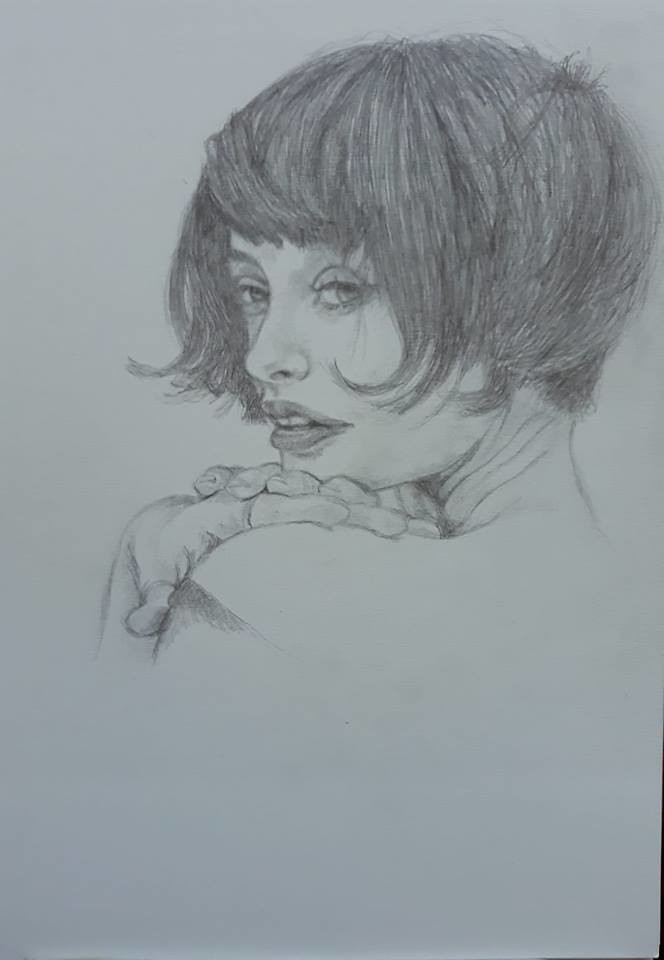This is a detailed pencil drawing rendered in black and white on a white piece of paper, slightly shadowed to a light gray. The drawing, occupying the upper two-thirds of a vertically oriented page, portrays a middle-aged woman with a striking sense of maturity, reminiscent of the 1920s era. Her hair is a short bob, just above chin-length, with bangs that frame her face. The hair, dark and shaded with pencil strokes to suggest motion, curls forward on the sides, falling just below her ears in a pixie cut style longer in front than in the back. 

The woman is depicted standing with her back to the viewer, her head turned to the left, capturing a three-quarter profile as she looks over her left shoulder. Her large, expressive eyes are open, framed by long eyelashes, and her lips are dark and slightly parted, revealing her top two teeth and a side view of her nose with one nostril. She rests her hands on her left shoulder, chin nestled atop them, creating subtle folds and wrinkles in her neck. The drawing fades out just below her shoulders, suggesting she might be unclothed, emphasizing her graceful, mature demeanor.